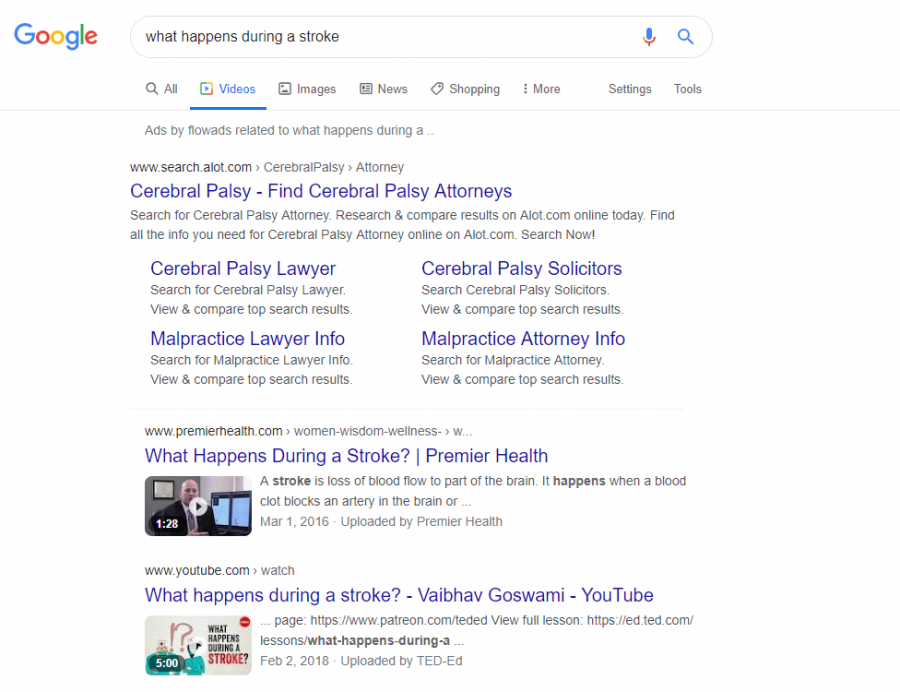In the upper left corner of the image, the distinctive Google logo is displayed in its traditional colors of blue, red, yellow, and green. Within the search bar, the query "what happens during a stroke" is visibly typed out. Just below this, the "Videos" tab is highlighted in blue, indicating that the search results are filtered to show video content.

The first search result appears with a link to www.search.alot.com. This link is followed by breadcrumb-style navigation: an arrow pointing right to "cerebral palsy," another arrow pointing right to "attorney," culminating in the clickable blue text "cerebral palsy – find cerebral palsy attorneys." Additional clickable links are listed underneath, including "cerebral palsy lawyer" in blue, "malpractice lawyer info," "palsy solicitors," and "malpractice attorney info."

Positioned below this initial result, there is a smaller, gray text that reads "premierhealth.com." This is accompanied by the description "what happens during a stroke." Adjacent to this description is a clickable video thumbnail that is 1 minute and 28 seconds in length, featuring a man in a suit positioned next to a computer screen.

Further down, another search result from youtube.com is shown with the thumbnail of a video titled "what happens during a stroke." The video thumbnail, lasting five minutes, prominently features the word "stroke" in red text followed by a question mark.